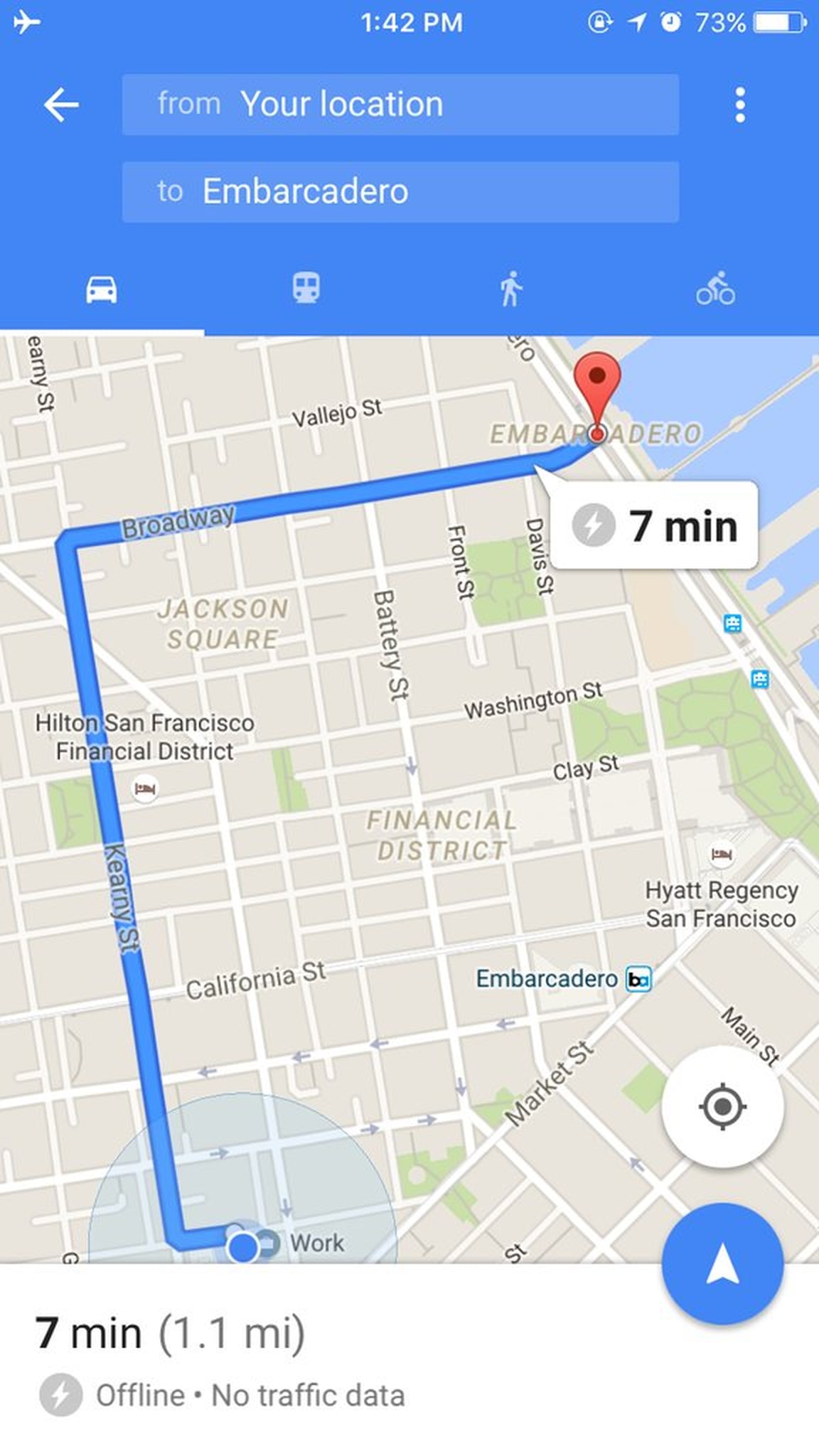### Descriptive Caption for Google Maps Image:

This image displays a screenshot from Google Maps, seemingly taken on a mobile device at 1:42 PM. The top of the screen features a blue status bar with a white airplane icon on the left, indicating the use of airplane mode. Centrally positioned, the time is displayed, and on the right side, the battery icon shows 73% charge, along with an alarm symbol and another icon indicating GPS and rotating lock status.

Below the status bar, the interface includes two light blue banners. The first banner, in white text, reads "From your location." Directly underneath, it specifies the destination as "To Embarcadero," with the text spelled out clearly. The right side of these banners features a vertical trio of dots, commonly used for additional options or settings.

Directly under the banners, a row of icons represents different modes of transportation: a white car, a bus or train, a person walking, and a person on a bike. A line appears under the car icon, signifying that the directions provided are for driving.

The map itself displays a segment of San Francisco, including notable landmarks such as the Hyatt Regency San Francisco and Tilton San Francisco Financial District. The route starts at the indicated position "Work," marked with a blue circle outlined in white. A thick blue line traces the recommended driving path, crossing Broadway and ending at Embarcadero. The destination is highlighted with a red location marker and a smaller red circle beneath it.

A prominent white banner has popped up on the map, stating "7 minutes" in bold black text, implying the estimated travel time. The lower part of the screen features standard navigation elements: a white circle with a black compass for directional orientation and a blue circle with a white arrow for initiating voice-guided navigation.

Further down, details on the travel time and distance are displayed: "7 minutes" in black text, with "1.1 miles" in gray parentheses, followed by a note in smaller text indicating "Offline. No traffic data."